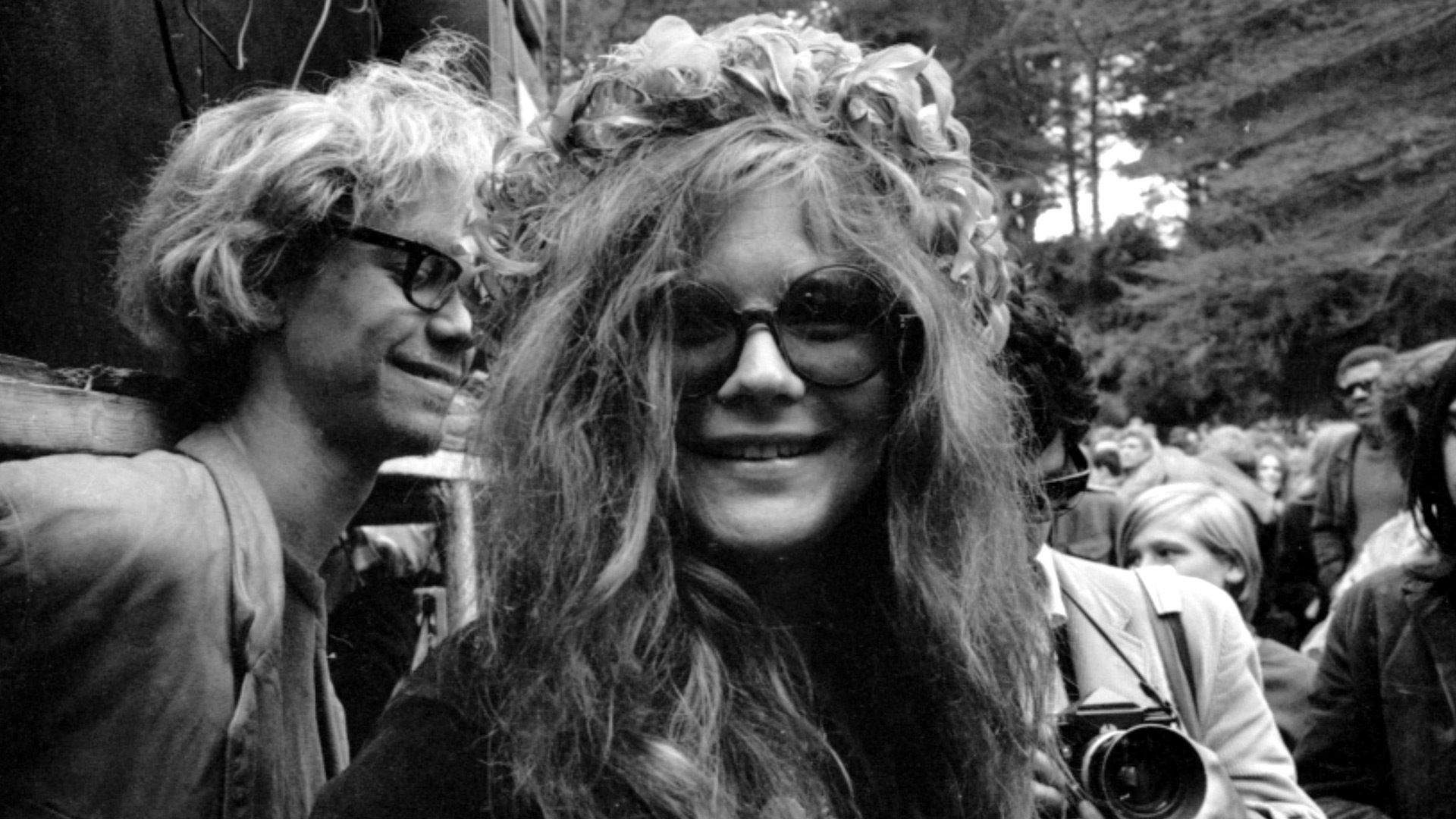This black and white photograph, likely from the 1960s, captures a moment of travel or participation in an event. Central to the image is Janis Joplin, the iconic singer, who is looking straight ahead and smiling while wearing round sunglasses and a black sweater. Her hair is partially up in a bun adorned with a ribbon, with the rest cascading beyond her shoulders. To the right of Janis (to the viewer's left), a man with short, almost bob-like hair and glasses is captured in profile, possibly blinking. He wears a buttoned-up suit jacket. The background features a crowd, suggesting a public event or parade setting. A camera held by the man appears over Janis's left shoulder, adding a layered depth to the photo. The overall scene exudes a retro, hippie vibe emblematic of 1960s counterculture.